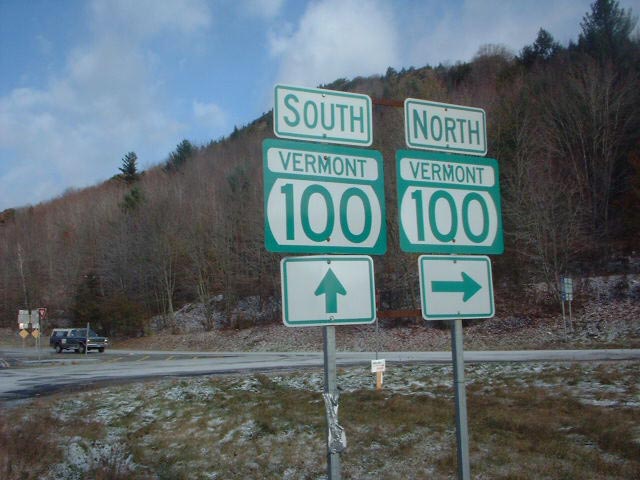The photograph captures a serene evening scene on a freeway, likely around 5 o'clock, with the sky transitioning towards dusk, adorned with a scattering of clouds. Prominently displayed in the center of the image are two green and white freeway signs mounted on a silver pole. The sign on the left reads "South Vermont 100" with an upward arrow indicating straight ahead. The sign on the right reads "North Vermont 100" with a right-pointing arrow. 

The backdrop features a picturesque mountainside adding a natural grandeur to the scene. Below the signs, a well-maintained asphalt road forms a three-way intersection, contributing to the orderly traffic flow. A black hatchback is stationary on the road behind the signs, appearing to pause perhaps at a stop sign or traffic light. Further adding to the realistic feel of the setting, additional street signs are visible around the intersection. The overall composition of the image conveys a tranquil yet utilitarian snapshot of everyday travel against the backdrop of natural beauty.